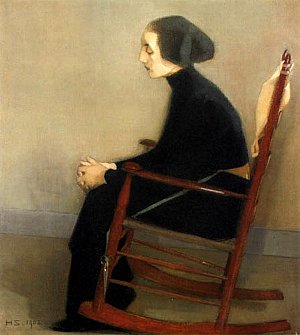The painting depicts a solemn woman seated in a wooden, reddish or mahogany-colored rocking chair, facing to the left side of the image. She wears a long black skirt and a black long-sleeved top, with a black head covering that suggests her hair is either pulled back or hidden under a netting. The woman sits with her arms crossed in her lap and eyes closed, conveying a pensive and mournful expression, as if she might have lost someone dear. Her face appears pale against the austere background of beige walls and a darker beige or brown floor. There is minimal decoration, with just a slight baseboard along the floor, enhancing the simplicity of the room. The bottom left-hand corner of the painting features the initials "HS" and the year "1881", indicating the artwork's historical context.